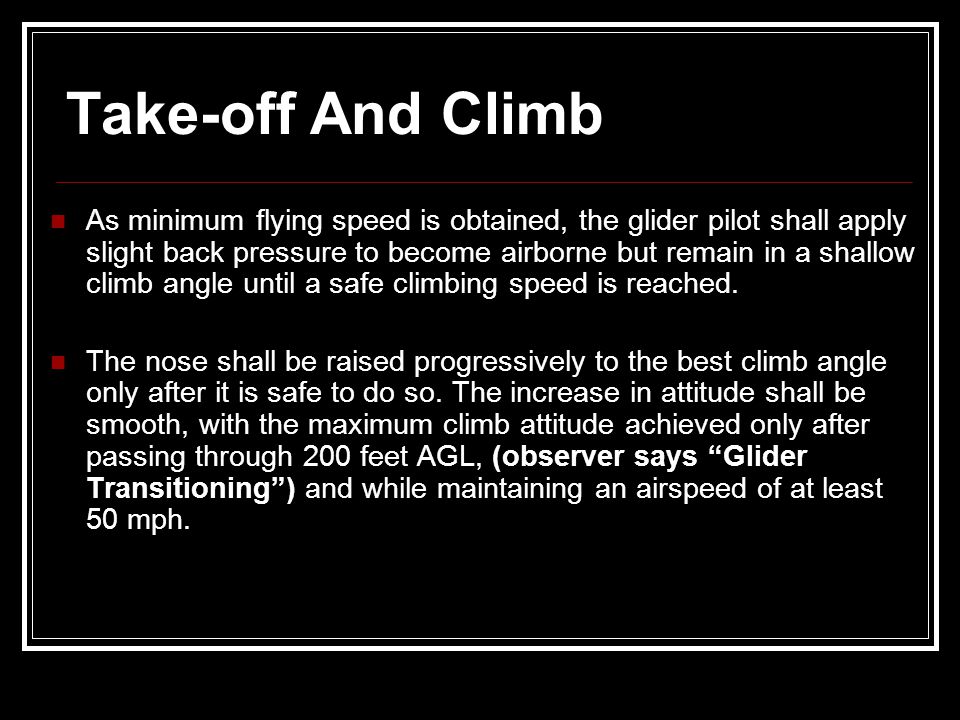The image is a detailed instruction slide that appears to be part of a presentation, possibly a PowerPoint. It features a black background with centered white text and a white border framing most of the image. At the top, a bold headline reads, "Take Off and Climb," followed by two bullet points in red with white text. These instructions detail that as the minimum flying speed is obtained, the glider pilot should apply slight back pressure to become airborne but maintain a shallow climb angle until a safe climbing speed is reached. It further advises that the nose of the glider should be raised progressively to the best climb angle only when it is safe, and the increase in altitude should be smooth, achieving maximum climb altitude only after passing 200 feet AGL. An observer note in bold parentheses states "Glider transitioning," emphasizing maintaining an airspeed of at least 50 miles per hour. Additionally, there is a notable red line underlining the top text, contributing to the organized presentation style of the slide.